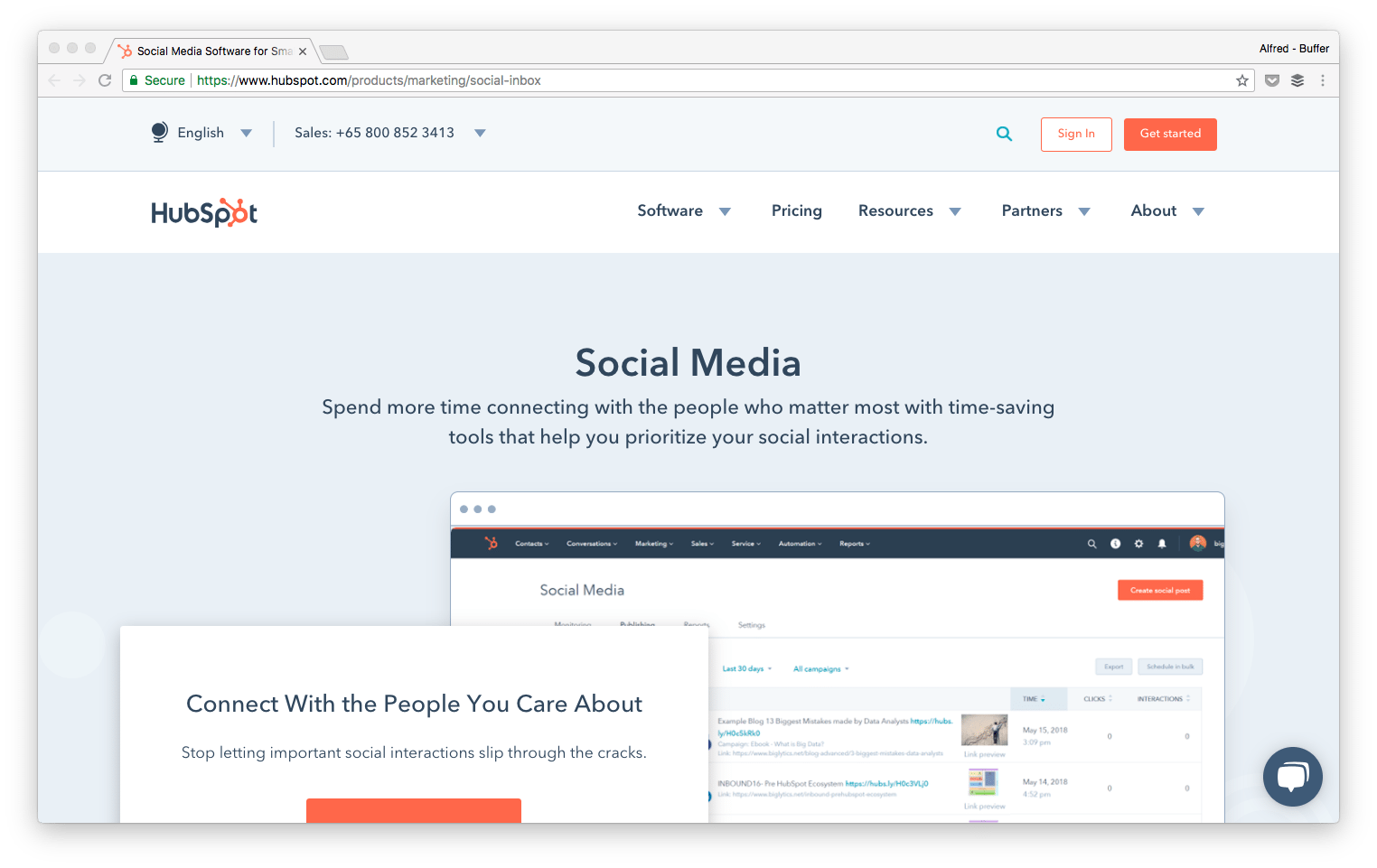A screenshot captured from the HubSpot website interface showcases a detailed web page layout. 

In the upper left, the background is a uniform gray with three gray dots indicating a customizable option or menu toggle. Below this, the browser tab reads “Social Media Software for...,” but the full text is not entirely legible. Adjacent to this tab, another tab appears labeled “Buffer” or something similar. 

The browser area features navigation buttons on the left, including grayed-out left and right arrows, and a grayed-out refresh icon. The URL bar displays the website address “www.hubspot.com” in black text, followed by supplementary gray text not fully articulated.

Further right in the address bar, several icon buttons are visible: a star for bookmarking, a peculiar shield icon perhaps for security or privacy settings, and a stack of three papers symbolizing documents or tabs.

Below the address bar, on the far left, a globe icon signifies language selection next to the text "English". Adjacent is a customer service number, "+65 800 85 234 13," accompanied by a drop-down menu.

On the extreme right of the interface, a magnifying glass icon allows for site search functionality. Nearby, a "Sign In" button and a contrasting "Get Started" button (white text on an orange background) are visibly prominent.

The main content area contains the HubSpot logo, primarily in black with a distinctive 'O' character. Below the logo, there are navigational links labeled "Software," "Pricing," "Resources," "Partners," and "About." A bold headline reads: “Social Media: Spend more time connecting with the people who matter most with time-saving tools.”

Two additional browser screens appear minimized at the bottom, while a blue messaging widget with two speech bubble icons hovers in the bottom right corner, suggesting customer support or chat functionality.

This detailed layout reflects a snapshot of a comprehensive digital interface from the HubSpot website.